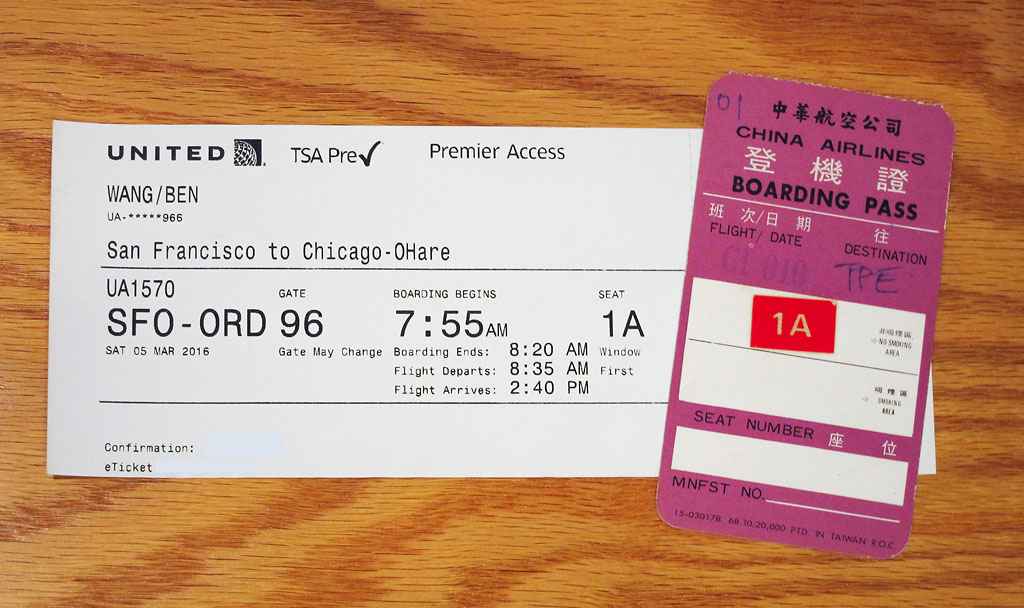The image features a horizontal rectangular receipt-like document laying on a medium brown, wood-grained table. This document appears to be a plane ticket from San Francisco to Chicago O'Hare Airport, prominently marked with various stamped information. Positioned over this ticket on the right side is a slightly tilted purple boarding pass. Key details on the white paper ticket reveal it is for United Airlines, flight UA1570, departing at 7:55 AM, with seat assignment 1A, and the passenger is Ben Wang. The date of the flight is identified as Saturday, March 5th, 2016. Additionally, the purple boarding pass belongs to China Airlines, for flight C1010 to TPE, also showing seat number 1A. The contrast between the white United Airlines ticket and the purple China Airlines boarding pass is visually striking against the wooden surface, with clear details such as the airline names, flight numbers, and passenger seat information.